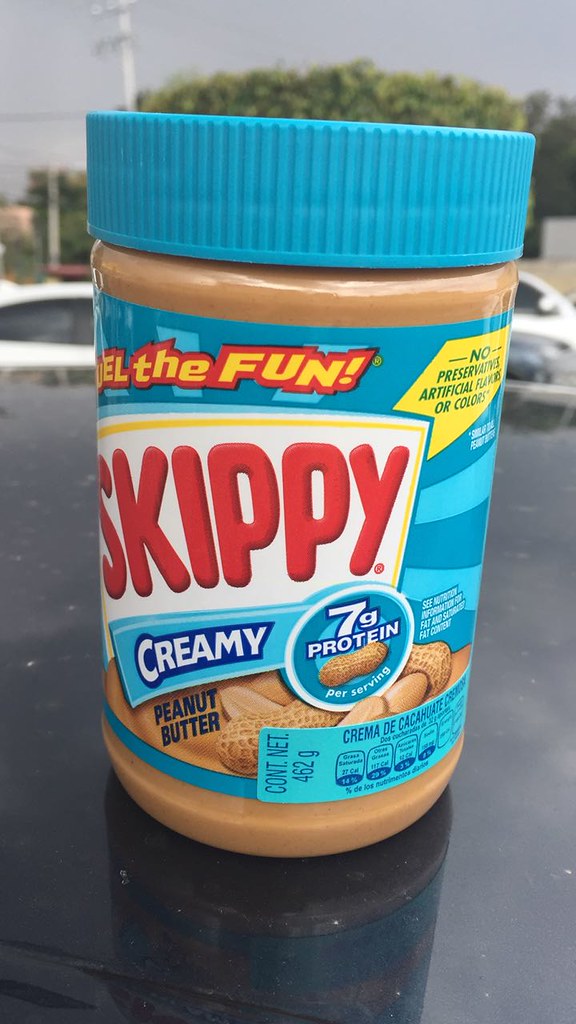This vivid color photograph provides a close-up view of a Skippy peanut butter jar, emphasizing its prominent branding and details. The jar, likely made of plastic, features a distinctive turquoise blue lid, a signature color for the Skippy brand. The familiar Skippy logo stands out prominently against a white label, written in bold red letters with "creamy" specified below it. Additionally, there is a circular insert highlighting "7 grams of protein." Below the word "creamy," the label indicates "peanut butter," complemented by an image of peanuts still in their shells. At the very top, above the white label, the partial slogan "the fun" is visible, though the rest of the phrase is obscured. The jar is positioned on a highly reflective, gray-colored table. The background reveals an outdoor setting, evidenced by a gray sky, green trees, and a partial view of a white car on the left side. This detailed environment enhances the focal point, the Skippy peanut butter jar, giving it context and a sense of place.